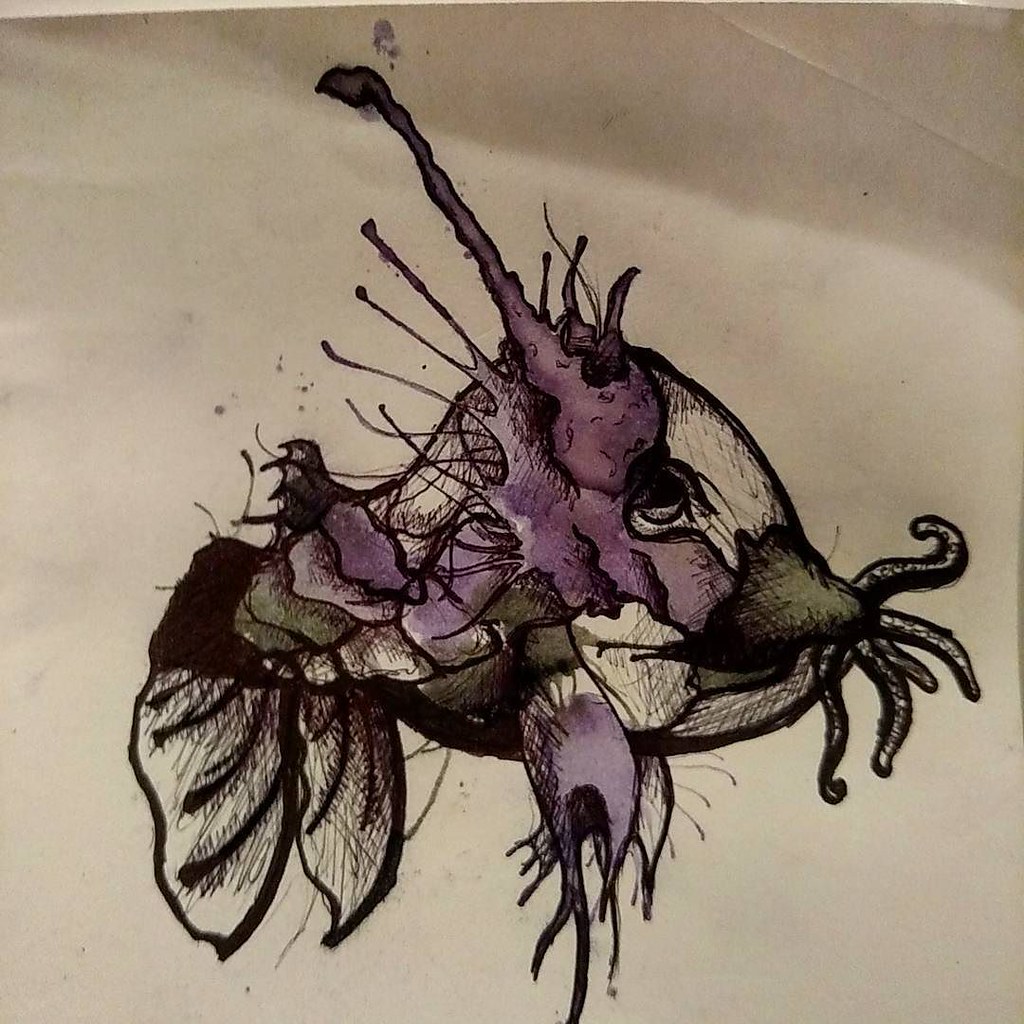This photograph captures a detailed watercolor painting that appears to be expertly crafted on a slightly beige, white canvas paper. The painting features an abstract and surreal creature that resembles a hybrid between a zombie fish and a catfish. The fish is predominantly defined by thick black outlines, suggesting the use of pen to sketch its form before adding watercolor. It is depicted facing towards the right and is viewed in profile, with its right eye clearly visible.

The fish exhibits a peculiar blend of colors including purples, greens, and browns, and its body is composed of numerous intriguing elements. Its gills are painted in a violet hue, and the mouth area showcases light green shades. Extending from its mouth are tentacle-like appendages that resemble worms or an octopus. Two back fins and two side fins adorn the fish, with the side fins uniquely resembling flower petals curving downwards. The creature also boasts a distinctive long, purple antenna or strand that protrudes from the top of its head, accompanied by several smaller antennae-like structures.

In the painting’s background, there are scattered purple paint spots, suggesting accidental drips, which add to the organic and spontaneous feel of the artwork. Additionally, the paper slightly curves inward towards the camera, subtly highlighting the texture and material of the canvas. The combination of exquisite detail and unusual subject matter underscores the artist's skill and creativity.